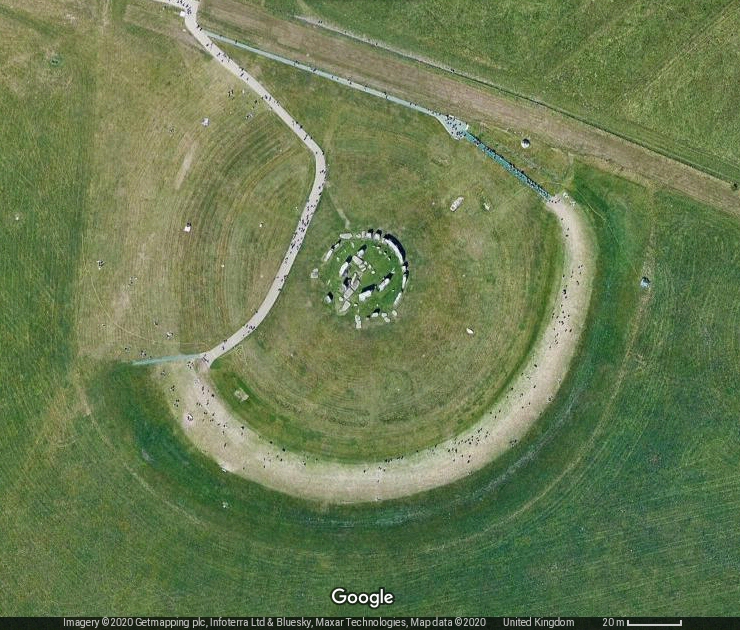This aerial photograph, likely taken by Google in 2020, depicts a countryside area in the United Kingdom. Dominating the center of the image is a vast circular formation, bordered by lush green grass. The circle consists of multiple concentric rings: the outermost green circle is followed by a white band, a lighter green ring, and finally a dark green core. Encircling the center within the dark green area are arrangements of stones reminiscent of Stonehenge, suggesting an ancient or historical site. A straight brown road traverses the upper segment of the image, while another white pathway meanders through the rings of the circle. The image includes a few indistinct dots which might represent people, indicating potential tourist activity. Surrounding the circle, the landscape is primarily green with open grassy areas, though a section of the ground appears brown due to soil exposure. The bottom of the photograph features the word "Google" in white font, and beneath it, a black horizontal strip displaying additional details and scale information.